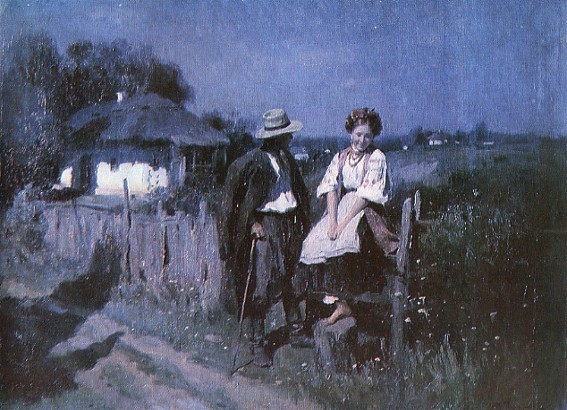This image is a detailed print of an old painting primarily rendered in dark tones with hints of deep blue in the night sky, which is dotted with a few stars. The central focus is a man and a woman. The woman, barefoot, sits on an aged wooden fence with one foot resting on a stump. She wears a dark dress with a white blouse and apron, and her hair is adorned with flowers. The man beside her is leaning on a cane, dressed in a gray hat, long black coat draped over his shoulders, gray slacks, and a white shirt. Behind them, the fence appears rickety, enclosing a yard filled with weeds and shrubbery. To the left, there is an old house characterized by its thatched roof and white walls, with a tree standing behind it. A dirt road with a grass strip down the center winds past the couple. In the distance, beyond the right side of the fence, a hill rises, crowned with another white house.